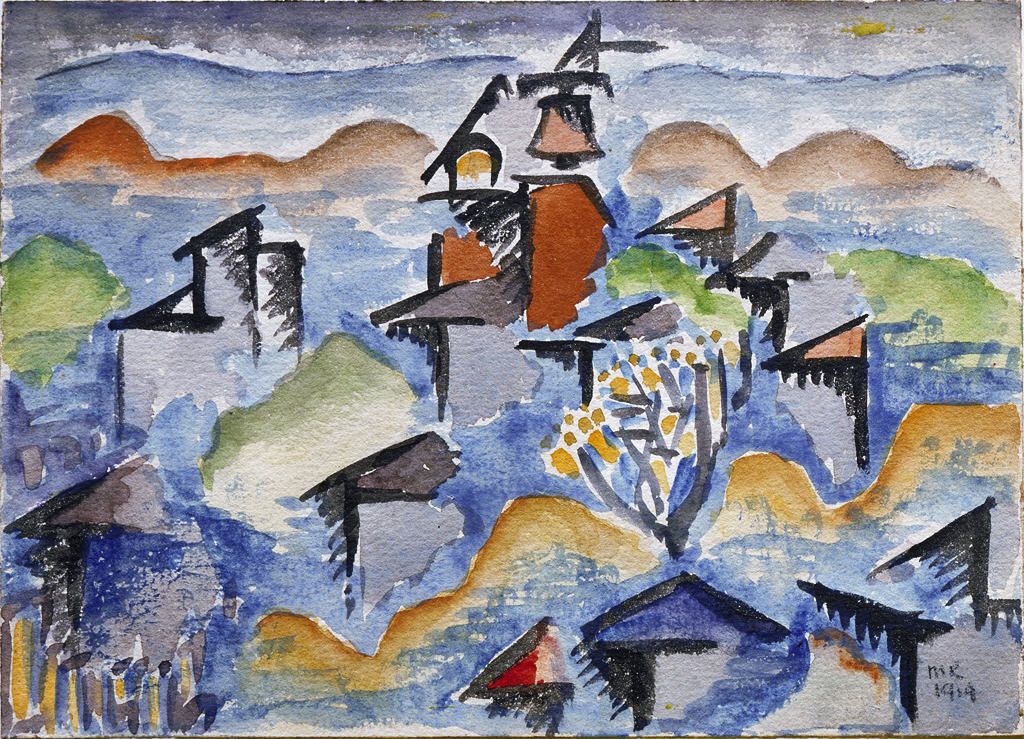The image features an abstract watercolor painting imbued with a multitude of vibrant colors, predominantly blue, with significant use of brown, black, green, yellow, and occasional red highlights. Principally, the image portrays an outdoor setting filled with fragmented representations of various buildings, outlined in black, some of which are taller than others. A prominent bell tower stands at the center, suggesting a focal point amidst the architectural array. Additionally, yellow and brown hues are utilized to depict hills or mountaintop areas in the background beneath a blue-grey sky with a sun appearing through clouds on the right-hand side. Green areas near the middle hint at grassy fields or trees, interspersed with a notable tree with yellow leaves in the foreground. A part of the painting bears the text "MK 1914" located in the blue-black lower right corner, adding a historical touch to this complex and colorful composition.